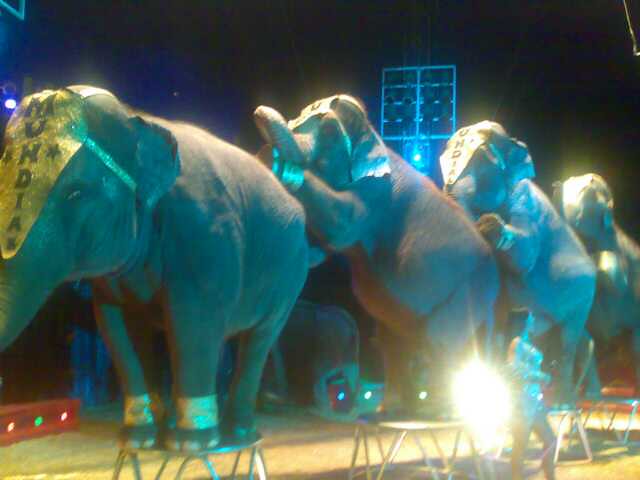The image captures a somewhat out-of-focus night scene at a circus, featuring a quartet of elephants performing a synchronized act. All four elephants face the left, with the foremost elephant standing with all four feet on a circular metal stool. This lead elephant is adorned with gold cuffs on its front ankles and a banner on its forehead. This banner has a gold background and the word "Mundia" written vertically in black letters, held in place by gold-colored straps. The subsequent elephants are positioned sequentially, each standing with their rear feet on a stool and their front feet resting on the hindquarters of the elephant ahead. Each elephant wears a similar forehead banner as the first. In the background, the circus lights illuminate parts of the scene, revealing a person in a silvery outfit with long black hair, possibly an entertainer. Silver tables circle the area, contributing to the ambient circus setup.